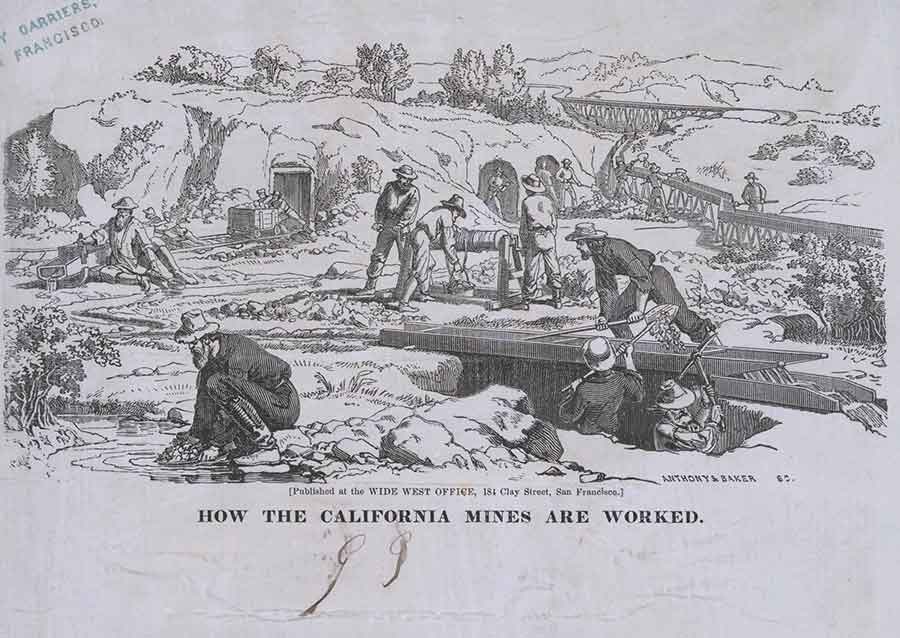This black-and-white drawing, set on light gray paper, illustrates an industrious scene of early California mine workers amidst a detailed natural landscape. The upper left-hand corner features partially visible text in green, including the words "carriers" and "Francisco," indicative of some incomplete caption. Prominently, the bottom of the page bears the title "How the California Mines Are Worked."

The composition is rich with activity: men, who are all wearing hats and long-sleeve outfits with long pants, are depicted engaging in various mining tasks. To the left, there's an entrance to a hillside mine, with railroad tracks extending from it. A man sits beside these tracks, observing others who operate a hoist or bucket nearby. Scattered across the scene are additional men using shovels and specialized tools, including sickle-like implements, indicative of the intensive labor involved.

Towards the right of the drawing, small bridges span a modest river, facilitating the movement of workers and materials. In the foreground, a couple of men stand in a pit while another man supervises from above. To the bottom left, a miner is engaged in panning for gold in a creek, surrounded by rocks and sparse vegetation. The background is dominated by mountains and trees, completing the rugged and determined atmosphere of this 19th-century California mining operation.